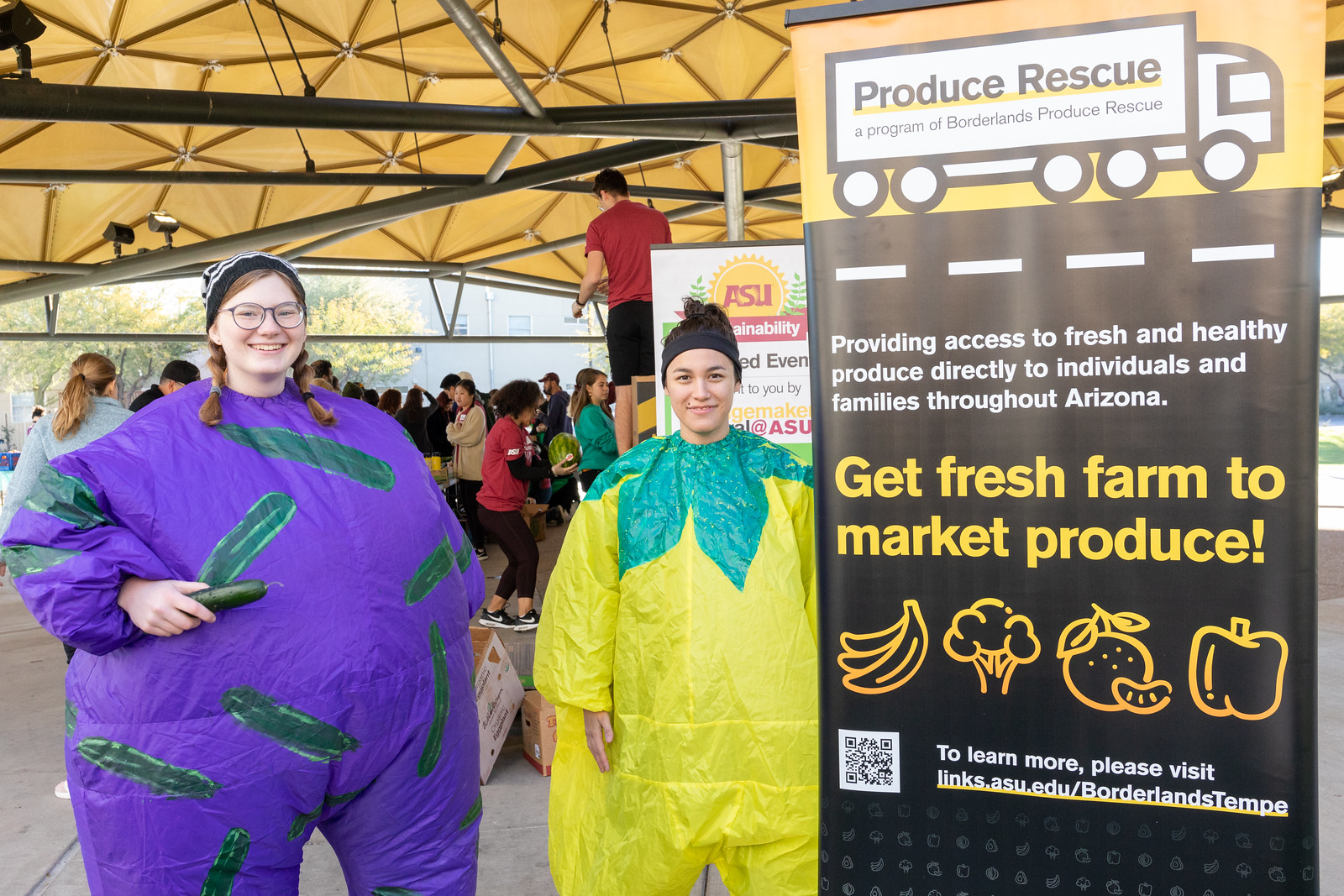The photograph features two women in colorful costumes standing in front of a large rectangular sign. The woman on the far left is dressed in an oversized purple suit adorned with cucumber illustrations, which makes her appear very large. She is wearing regular glasses, a black and white beanie, and has her red hair styled in pigtails. She is also holding a cucumber in her right hand. Next to her on the right is another woman wearing a yellow costume with green leaves around the neck, resembling a lemon. She is wearing a black neck cap. 

To the right of the women stands a tall, prominent sign. The upper part of the sign has a yellow background featuring a stylized black and white image of a truck. The truck has the words "Produce Rescue, a program of Borderlands Produce Rescue" written on its side. Below this, the sign is predominantly black with multiple sections of text and illustrations. The white text reads, "Providing access to fresh and healthy produce directly to individuals and families throughout Arizona." This is followed by yellow text stating, "Get Fresh Farm to Market Produce," and yellow line drawings of various fruits and vegetables, including a bunch of bananas, a head of broccoli, a single orange, and a bell pepper. There is also a QR code with instructions in white text that read, "To learn more please visit links.asu.edu forward slash Borderlands Tempe." In the background, a crowd of people and a white, yellow, or orange awning can be seen.